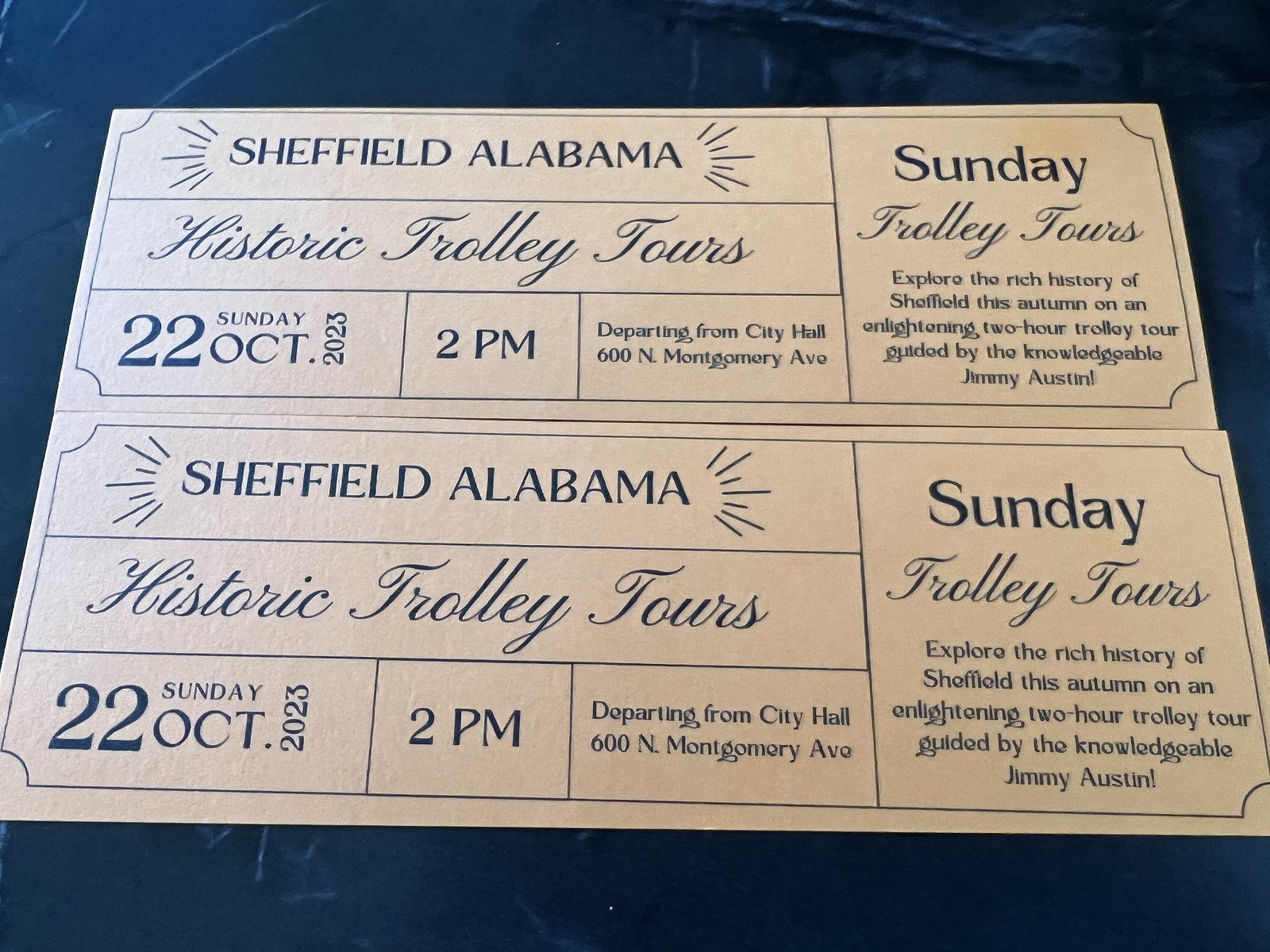This image displays a cream-colored poster with dark blue text. At the top, it reads "Sheffield, Alabama" followed by the cursive title "Historic Trolley Tours." Below that, the details are listed: "22nd October 2023, Sunday, 2 p.m.," along with the departure location, "City Hall, 600 North Montgomery Avenue." Next to this main section, on the right-hand side, another column repeats the event details, starting with "Sunday Trolley Tours." This section invites readers to "Explore the rich history of Sheffield this autumn on an enlightening two-hour trolley tour guided by the knowledgeable Jimmy Austin." The same information is reiterated below. The design is simple yet informative, with a clear emphasis on the historic and guided nature of the tour.